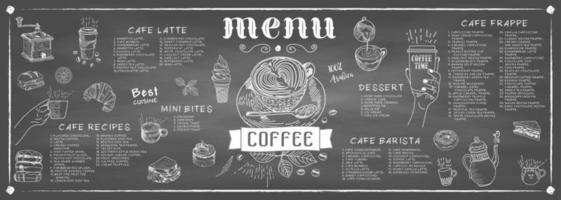The image features a professionally designed coffee menu set against a blackboard-like background with white chalk-style illustrations and text. The menu is long, rectangular, and bordered by a thin white line, with a small diamond shape at each corner. Central to the menu is an intricate chalk drawing of a latte art in a cup, placed on a saucer with a spoon beside it. Above the cup, the word "MENU" is prominently displayed, while a banner below the cup reads "coffee," flanked by small leafy designs.

Throughout the menu, different sections with labeled headings such as "cafe," "cafe latte," "mini bites," "cafe recipes," "best cuisine," "dessert," "cafe barista," and "cafe frappe" are displayed. The text is uniformly white, contrasting with the black background. There are detailed drawings of various coffee-related items and desserts, including a scone, an ice cream cone, a to-go cup labeled "coffee time," a coffee grinder, sandwiches, and a kettle. The artistry and monochromatic palette give the menu a cohesive and eye-catching appearance.